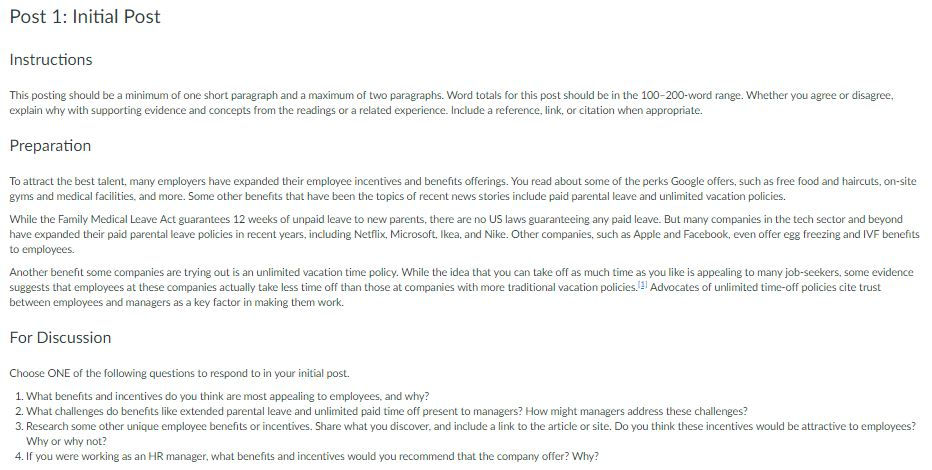The image displays an all-white background with black font text starting from the upper left corner. The text details the initial post instructions for an assignment, which should be a minimum of one short paragraph and a maximum of two paragraphs, with a word count between 100 and 200 words. The content must indicate whether the writer agrees or disagrees with the given statement and explain their stance with supporting evidence and concepts from the reading or personal experience, including a reference link or citation when appropriate. 

Beneath these instructions, the text discusses the strategies employers use to attract top talent, citing expanded employee incentives and benefit offerings. Examples include Google's renowned perks such as free food, on-site haircuts, gyms, and medical facilities. Additionally, contemporary benefits spotlighted in recent news, such as paid parental leave and unlimited vacation policies, are mentioned. Despite the Family Medical Leave Act guaranteeing 12 weeks of unpaid leave to new parents, the US has no law mandating paid leave. Nonetheless, many tech companies and others have enhanced their paid parental leave policies, with notable examples being Netflix, Microsoft, Ikea, and Nike. Employers like Apple and Facebook even offer advanced benefits such as egg freezing and IVF to their employees.